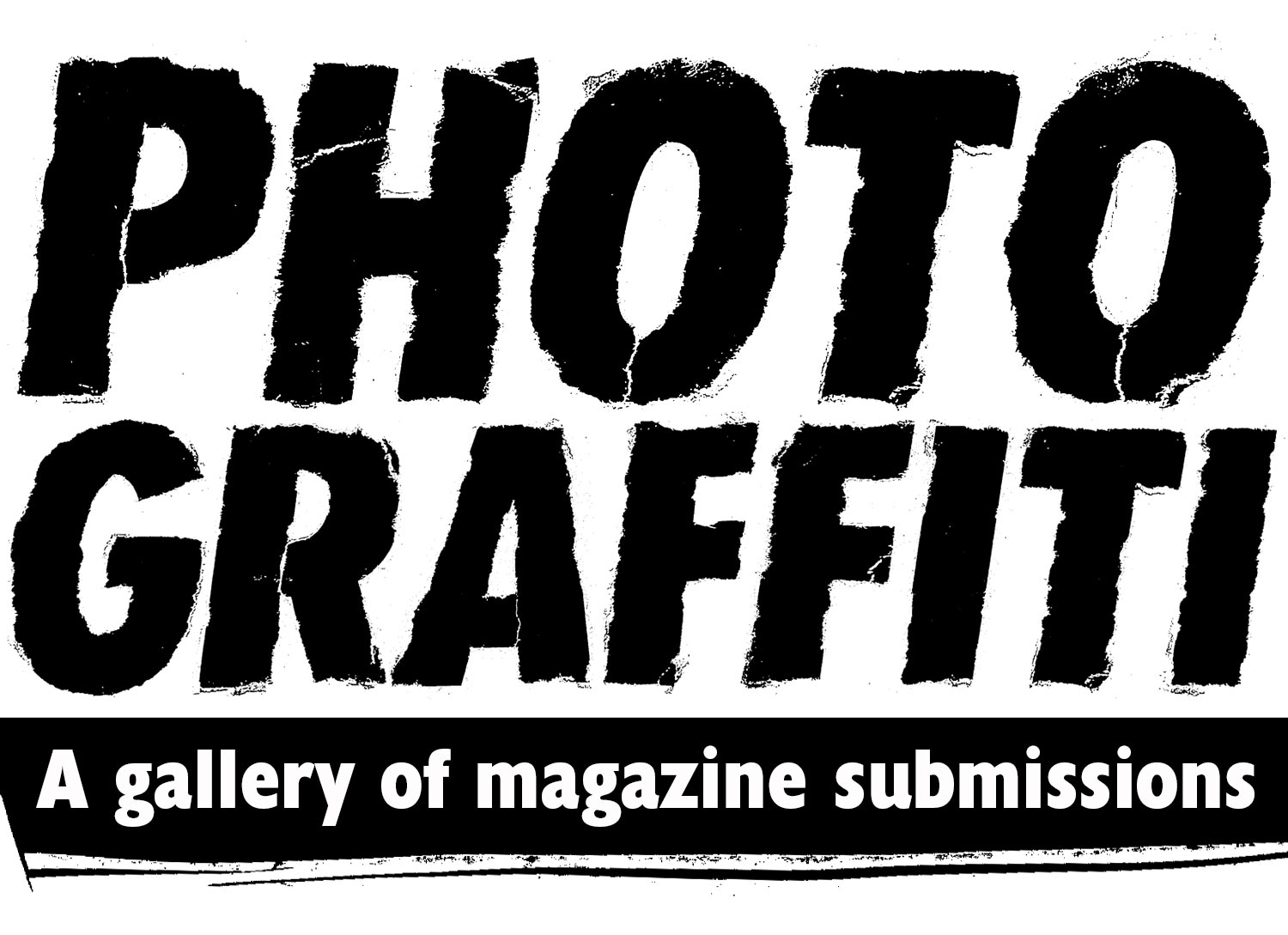A minimalist black-and-white image features bold, capitalized text that reads "PHOTO GRAFFITI" across the top. This heading, rendered in black against a white background, exhibits a distressed, rough texture with irregular lines and edges. For example, the letter "P" has an extended line descending from its interior loop, while the "H" has a subtle white line at its top-left and bottom-right corners. Both "O"s display lines running from their centers to their bases, and "R" mirrors the irregularity seen in the "P". Beneath this title, a clean-cut black box is centered, containing the phrase "A GALLERY OF MAGAZINE SUBMISSIONS" in crisp white lettering. Completing the design, a jagged black line is positioned below the box, adding an additional element of visual texture to the composition.